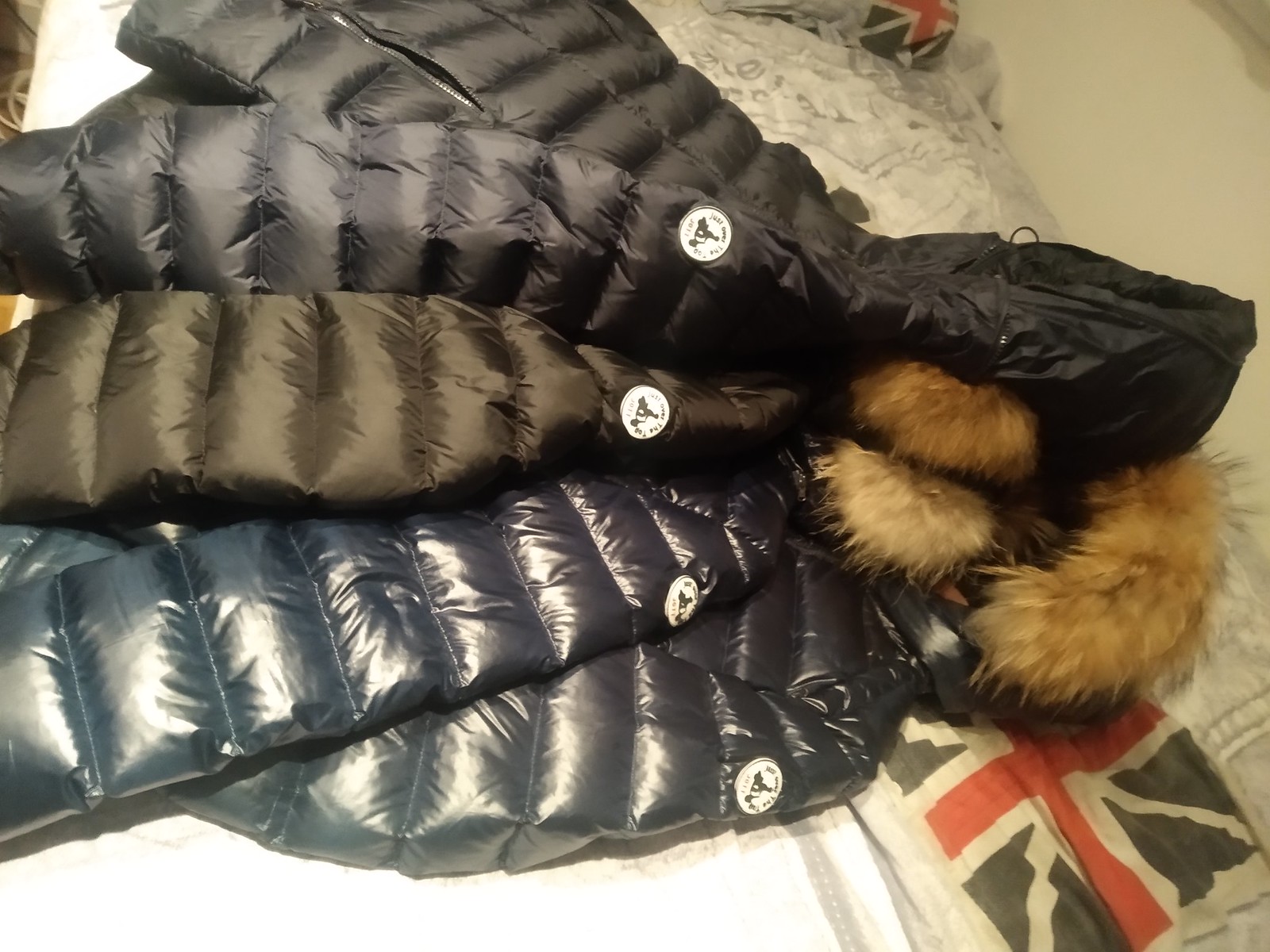This image features four winter puffer coats neatly laid out on what appears to be a gray and white, geometrically patterned bedspread, possibly made from a fabric that resembles denim. The bedspread is adorned with a prominent British flag (Union Jack) in the bottom right-hand corner, and another smaller flag just above and slightly to the left. Each coat, crafted from nylon, showcases its left-hand sleeve facing upward, revealing a round, black-and-white patch logo, though the text on the logo is indiscernible. The coats vary slightly in color: the one furthest up is black, followed by a dark brown, then a dark blue, and the one closest to the bottom is a dark gray. Three of the coats feature hoods rimmed with tan and brown fur trim, while one does not. There is a visible plastic zippered pocket on one of the coats, adding a functional detail to the winter ready ensemble.